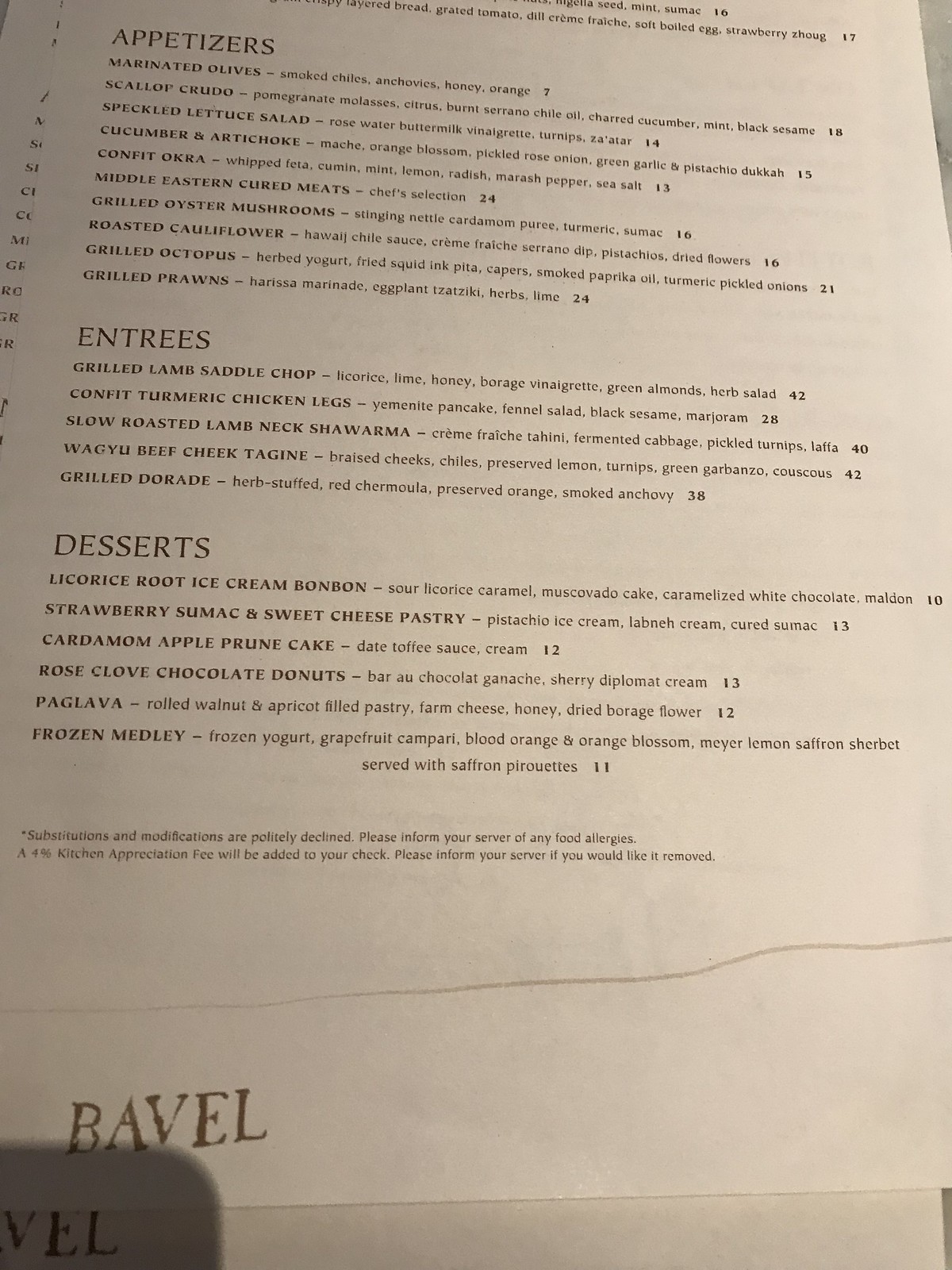The image depicts a comprehensive and gourmet restaurant menu categorized into appetizers, entrees, and desserts. 

**Appetizers:**
- Marinated Olives
- Scallop Crudo
- Speckled Lettuce Salad
- Cucumber and Artichoke 
- Confit Okra
- Middle Eastern Cured Meats 
- Grilled Oyster Mushrooms 
- Roasted Cauliflower 
- Grilled Octopus 
- Grilled Prawns 

**Entrees:**
- Grilled Lamb Saddle Chop
- Confit Turmeric Chicken Legs
- Slow Roasted Lamb Neck Shawarma
- Wagyu Beef Cheek Tangent
- Grilled Dorade

**Desserts:**
- Licorice Root Ice Cream Bonbon
- Strawberry Sumac and Sweet Cheese Pastry
- Cardamom Apple Prawn Cake
- Roast Clove Chocolate Donuts
- Paglava 
- Frozen Medley

The menu offers a rich variety of flavors and ingredients, showcasing an array of meticulously crafted dishes that cater to diverse palates, from the savory magic of grilled octopus and lamb shawarma to the sweet indulgence of clove chocolate donuts and exotic paglava.